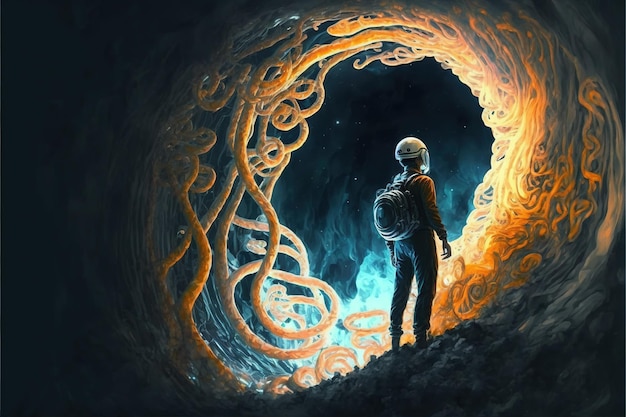In the digital artwork, a sci-fi traveler stands within a dimly lit tunnel, seemingly made from a combination of stone and intertwined, rope-like orange and white tendrils that curve and swirl around the opening. The figure is dressed in long sleeves and pants and wears an orange shirt over which a white helmet with a face shield and a backpack featuring a glowing yellow window can be seen. The darkened left edge and bottom corner of the image add to the overall ambiance of emerging from a shadowed cave. Ahead, an ethereal night sky filled with stars and a gradient of blue flames, from dark blue at the top to light blue at the bottom, illuminates the scene, casting an otherworldly glow.